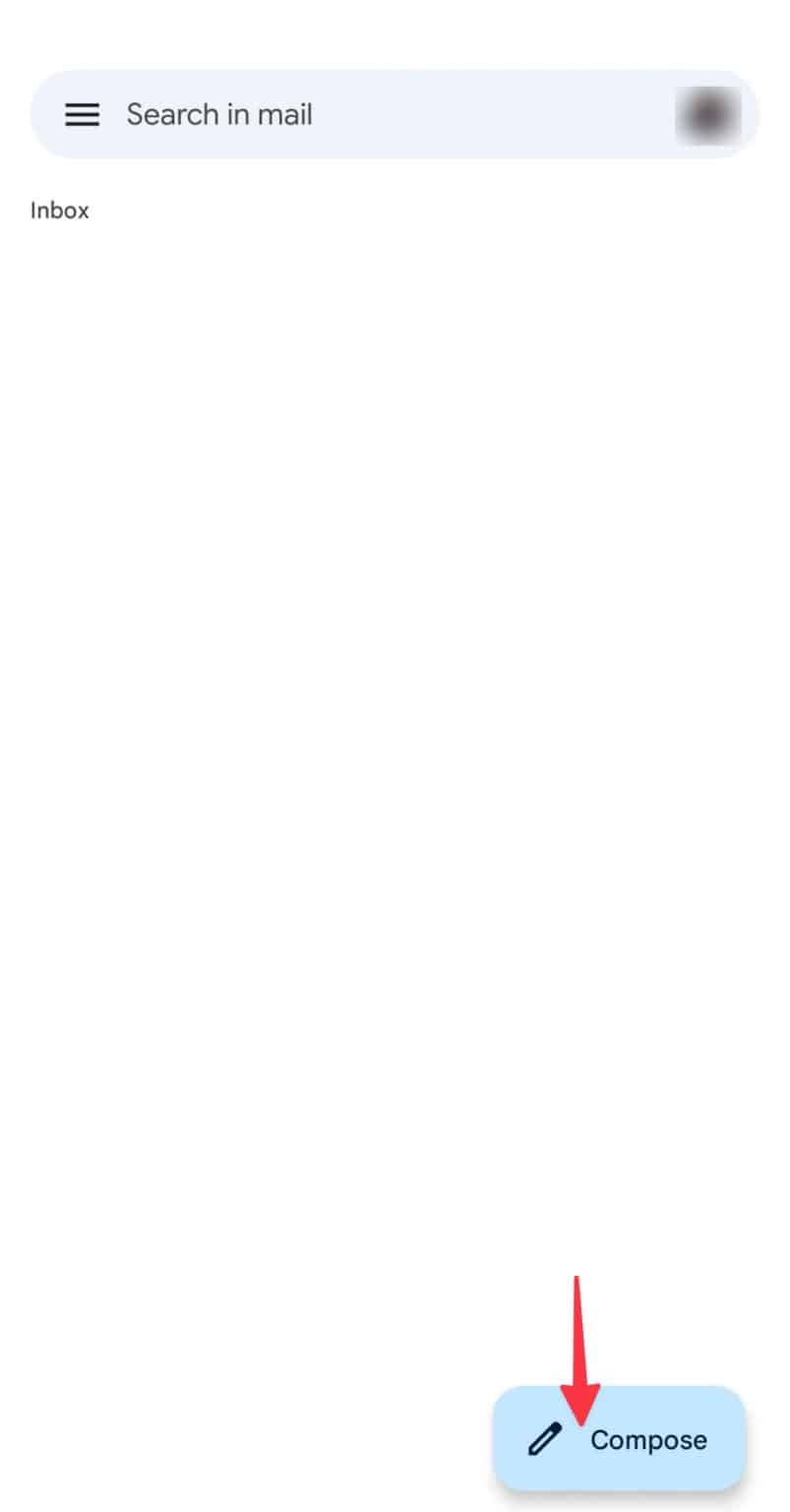The image depicts an email interface, characterized by its minimalist design and prominent user guiding elements. 

At the top of the screen, there is a gray, long oval-shaped search bar with a magnifying glass icon on the left side, followed by the text "Search in mail". To the right of the search bar, an icon appears to be blurred, suggesting it could be a user profile picture that is currently obscured or anonymized.

Below the search bar, the heading "Inbox" is displayed in a delicate, black font, matching the typographic style of the "Compose" button text. Notably, the inbox area is entirely empty, indicating that no emails are currently visible or loaded in this view.

Toward the bottom of the screen, a red arrow points to a prominently featured "Compose" button. This button is rectangular and baby blue, with a pencil icon next to the word "Compose," which is written in capital C and a refined font. The pencil icon includes a blacked-out end, representing the eraser.

The overall interface design is clean and straightforward, primarily using black font for text and neutral colors for icons, accentuated with minimal color highlights to direct user attention.